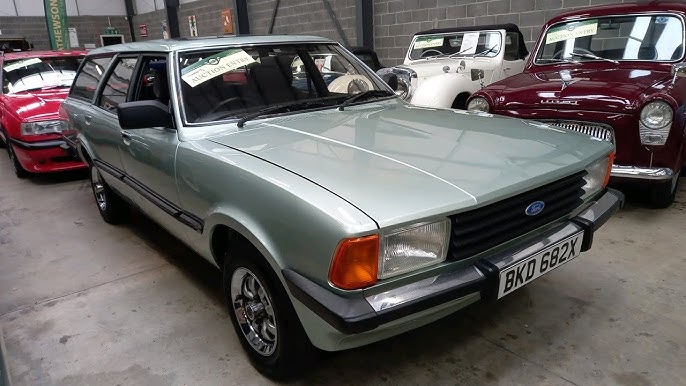The image depicts the interior of a garage-like car auction setting with unpainted cinder block walls that are gray, topped with white sections above. The floor is made of gray concrete. The central focus is on a shiny silver Ford station wagon with a white license plate bearing black letters "BKD 68 2X," suggesting it might be from another country. This Ford, an older model, slightly faces the right side of the image. In the background, several classic cars are visible, including a burgundy car from the 1970s and a white rounded sports car with a black convertible top. Behind the station wagon, the front end of a pinkish-red car is partially visible. Each vehicle has an auction entry sticker placed in the upper left corner of their windshields when viewed from the front, indicating their readiness for auction.